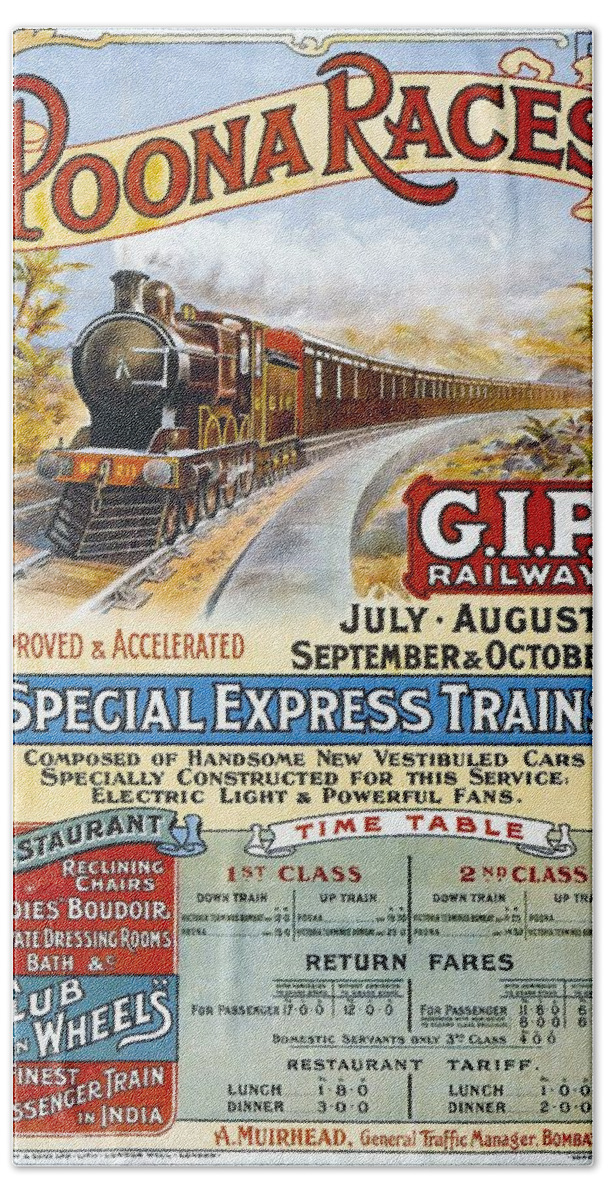This image is a vintage portrait-oriented advertisement for a special express locomotive train, promoting the "Puna Races" at the top. The train, an elegant old-fashioned model, is depicted making a turn amidst a natural setting. The text on the advertisement markets the "GIP Railway" for the months of July, August, September, and October, highlighting the train's improved and accelerated service. It boasts handsome new vestibule cars, electric lighting, powerful fans, and reclining chairs. Additionally, the ad describes a luxurious onboard experience, including a restaurant with reclining chairs, a ladies boudoir with dressing rooms and a bath, and a "club on wheels." The fares for first and second class, both for the down train and up train, are listed, albeit partially unreadable. The ad is signed off at the bottom by Mirrorhead, the General Traffic Manager.